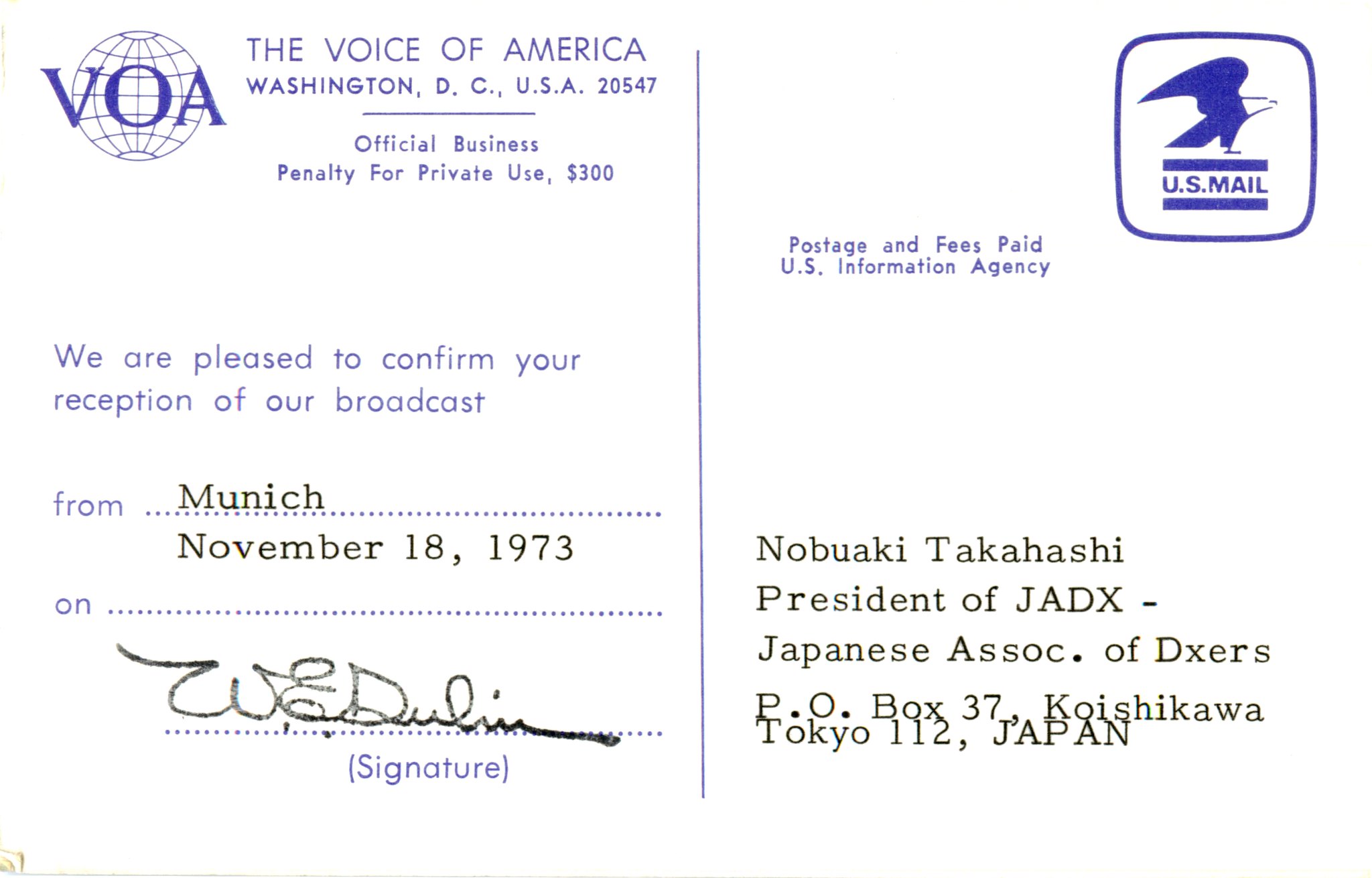This image showcases the back of a postcard from the Voice of America, Washington, D.C., USA, 20547. The top left features the VOA's logo alongside the text "Voice of America, Washington DC USA 20547, Official Business, Penalty for Private Use $300." Below this, the postcard reads, "We are pleased to confirm your reception of our broadcast from Munich, November 18, 1973," followed by a signature. On the top right, where a stamp would typically be, there is the U.S. Mail logo featuring an eagle, with the inscription "Postage and Fees Paid, U.S. Information Agency." The recipient's details are inscribed below: "Nobuaki Takahashi, President of JADX, Japanese Association of DXers, P.O. Box 37, Koishikawa, Tokyo 112, Japan." The postcard's background is white, with the text and icons primarily in blue and black colors.